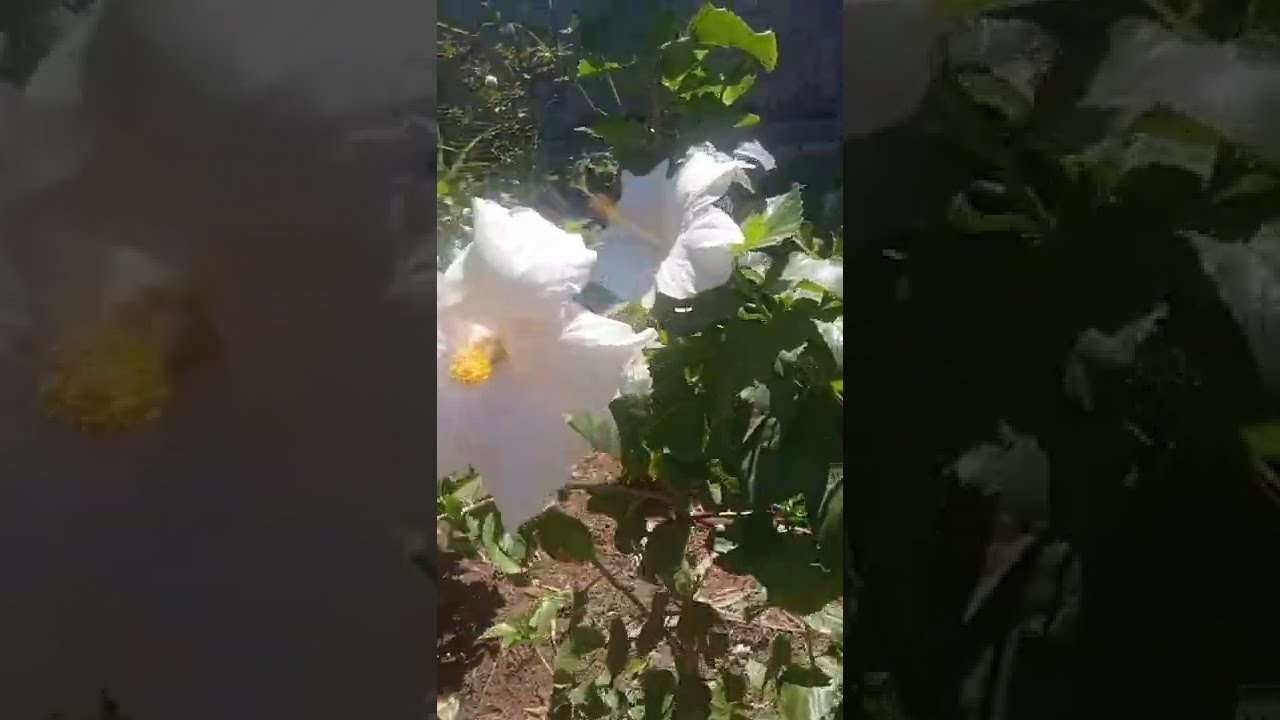In the center of the image, there is a close-up photograph of two white hibiscus flowers with about five or six petals each, showcasing their bright yellow stamens at the center. These flowers are part of a bush or large-stemmed plant with green leaves and a brown woody stalk. Sunlight bathes the flowers and surrounding scruffy green vegetation, while the simple dirt floor of the garden is visible beneath. The camera angle is slightly downward, capturing the flowers prominently. The image is framed by a zoomed-in and faded version of the same photograph, with the left panel featuring an enlarged close-up of one of the white flowers in lighter gray tones, and the right panel highlighting an even more detailed section of the green leaves against a darker, almost black, background.